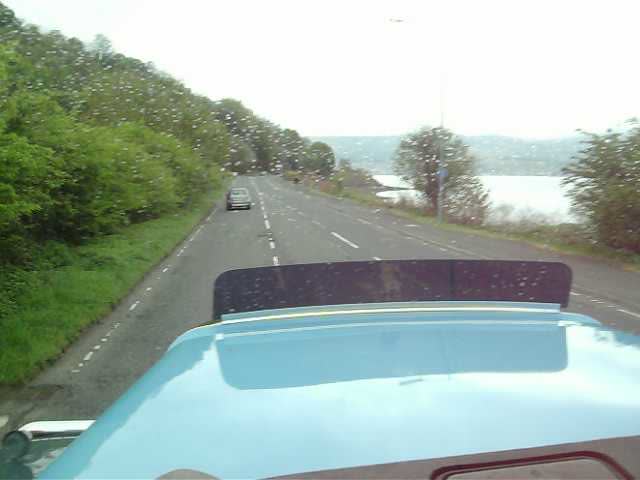The image captures a scene viewed from inside a vehicle, looking out the rear window. The vehicle has a light blue, possibly powder blue, shiny surface visible in the bottom part of the photo, indicating it might be the trunk or the hood. This smooth, metallic area matches descriptions suggesting it could belong to a truck or car. The road stretches ahead, appearing to be a four-lane highway divided by white dashed lines, with only one other visible vehicle far behind in the leftmost lane, distinguished by its very pale, grayish color. To the left, dense trees or thick bushes line the roadside, while to the right, a waterway can be seen, suggesting a scenic drive near a hill and a lake. The sky above is overcast, casting a white hue, with raindrops occasionally splattered on the windshield, highlighting the damp, reflective nature of the scene.